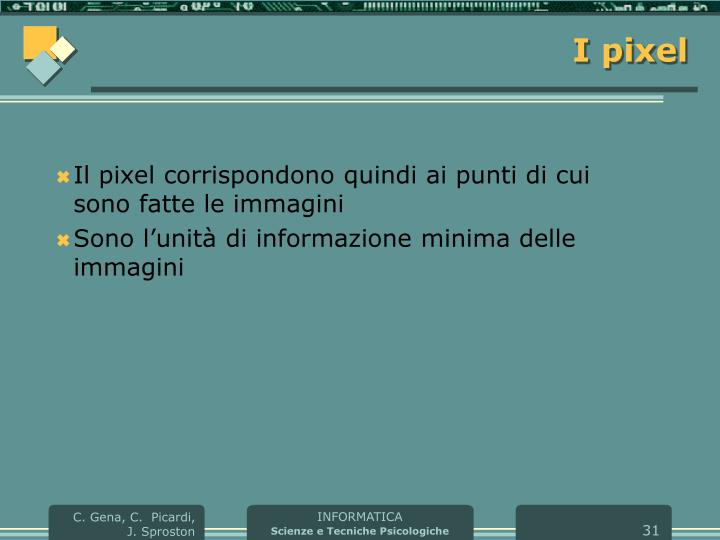The image is a computer screenshot with a dark teal background, featuring a green slide with white symbols and lines at the top. In the upper left-hand corner, there are three overlapping shapes: a large golden square, a tilted mint-green square, and a pale yellow square. On the top right-hand corner, "IPIXEL" is written in yellow letters. The center of the slide includes two bullet points marked by golden crosses. The first bullet point reads "IL PIXEL CORRISONDONO QUINDI AI PUNTI DI CUI SONO FATTE LE IMMAGINI," and the second one says "SONO L'UNITÀ DI INFORMAZIONE MINIMA DELL'IMMAGINI," both in black font. At the bottom of the slide, there are three dark green, rounded rectangles. The leftmost rectangle displays the names "C. GINA, C. PICARDI, and J. SPROSTEN" in white font. The middle rectangle reads "INFORMATICA" with "SCIENZE E TECNICHE PSICOLOGICHE" in smaller font underneath. The bottom right rectangle has the number "31," indicating this is the thirty-first slide of a presentation.